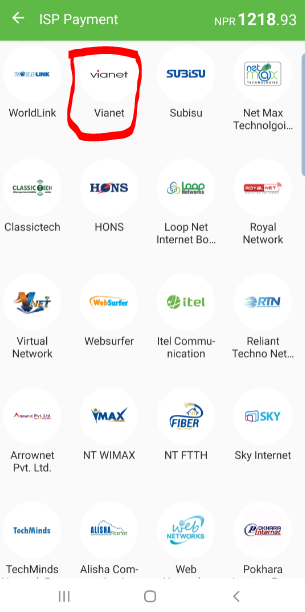This image is a screenshot of a pop-up window on a cell phone, characterized by its dimensions that mimic a mobile screen. The interface features a vivid green bar at the top with white text. On the left, there's a back arrow, followed by the label "ISP Payment." To the far right, the display shows "NPR" and a bold figure "121893."

Beneath the green bar, a white background displays a grid of ISP providers arranged in five rows and four columns. Each provider is accompanied by its respective logo. The providers listed from left to right in the top row are WorldLink, Vionet, Subisu, and NetMax Technologies. Vionet is prominently marked with a thick, crude, red marker circle.

The second row lists Classitech, Hans, LoopNet, and Royal Network, while the third row contains Virtual Network, WebSurfer, Intel Communication, and Reliant TechnoNet. The fourth row includes Arronet, NT-WiMAX, NT-FIS, and Sky Internet. The final row displays TechMinds, Aliciacom, Web, and Pokar.

At the bottom of the screen, three vertical gray lines, a gray square in the center, and a gray back arrow on the right complete the interface design.